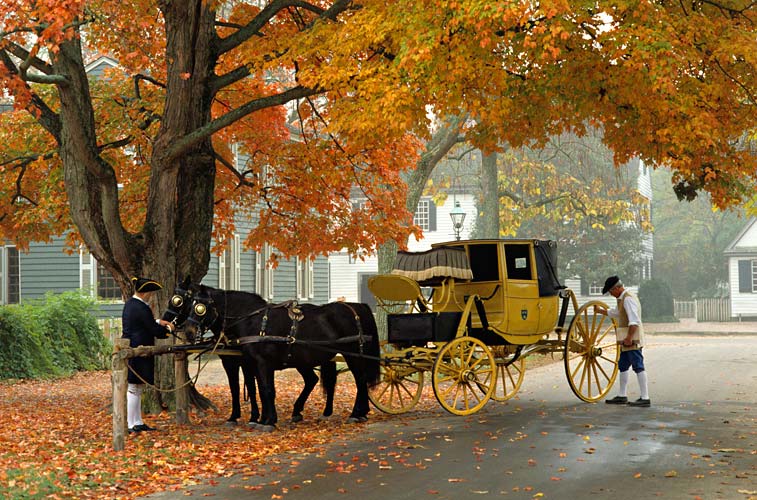In this highly detailed, color photograph set in an autumnal scene, we observe a captivating historical recreation in what appears to be a New England village. Dominating the left side of the image is a large oak tree, its branches laden with vibrant orange and yellow leaves, some of which have carpeted the ground below in a colorful display. 

Beneath this tree and next to an empty road stands a vintage yellow horse-drawn carriage, distinguished by its enormous wagon wheels and adorned with gray curtains. This nostalgic carriage, evocative of the mid to late 1800s pioneer times, is pulled by two black horses, each equipped with blinders. 

On the right-hand side of the carriage, near the largest wheel, a man in a white and blue colonial outfit and small black hat carefully examines the wheel, adding to the historic charm of the setting. Another man, dressed in a tricolor cap and colonial attire of a black suit with white trousers, stands to the left of the horses, feeding them over a small wooden fence. 

The scene is completed in the background by a grayish-blue colonial house partially obscured by the oak tree, a large white colonial house beyond that, and a quaint cottage off to the right. The entire tableau not only captures the essence of a bygone era but is also set against the breathtaking backdrop of autumn foliage, blending historical recreation with natural beauty.